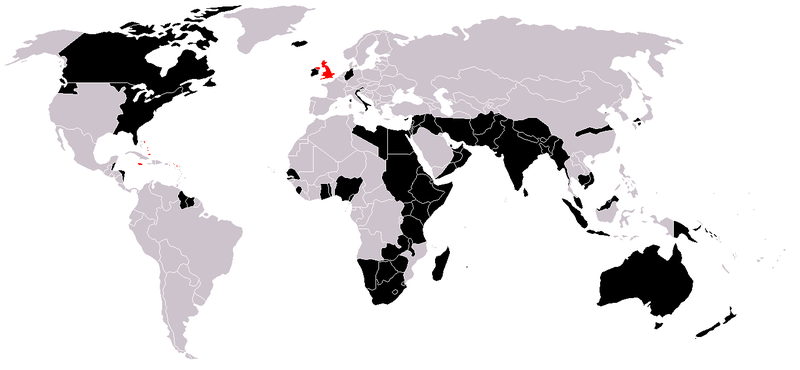This image features an animated map showcasing six of the seven continents: North America, South America, Asia, Africa, Europe, and Australia, with Antarctica not depicted. 

- North America is depicted on the far left, characterized by a half-black, half-light gray coloring.
- Directly below North America, and slightly to the right, is South America, which is predominantly light gray with a notable black patch at its northern end.
- Moving to the right, Africa comes next, also split into half black and half light gray.
- Above Africa lies Europe, which is mostly light gray with a distinctive red section and a few black spots.
- To the right of Europe is Asia, similarly light gray, but with its southern part colored black.
- Finally, in the bottom right corner, Australia appears, entirely colored in black. 

This visual arrangement effectively highlights the geographical positions and distinct color codings of these six continents.